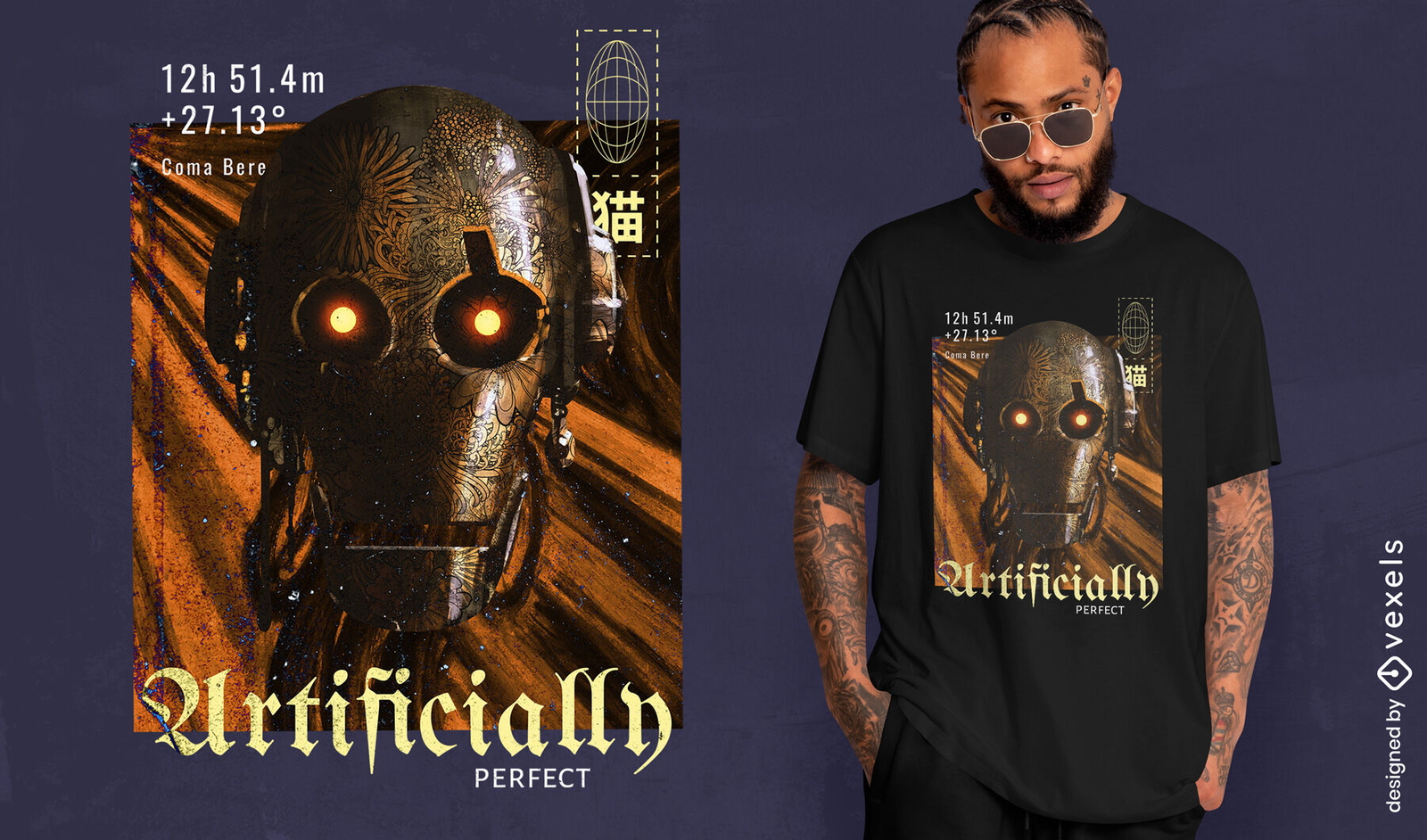The image features a promotional layout, possibly for a hip-hop or rap album. On the left side, there is an album cover displaying a robotic or skeleton-like head with glowing yellow eyes, reminiscent of a character from the new Star Wars trilogy. The cover includes text at the top left corner stating "12 hours, 51.4 minutes," "plus 27.13 degrees," and "coma, bury." Below these coordinates, it reads "artificially perfect" with a stylized "U". 

To the right of the album cover, there is an African-American man with short cropped hair, a beard, and mustache. He is wearing a black t-shirt featuring the same robotic image from the album cover. The man, donned in sunglasses, is looking outward, and his arms are adorned with tattoos. The background of the image is a grayish-blue hue. Text on the lower right side of the picture reads "decide by Vexels" or "copyright Vexels."